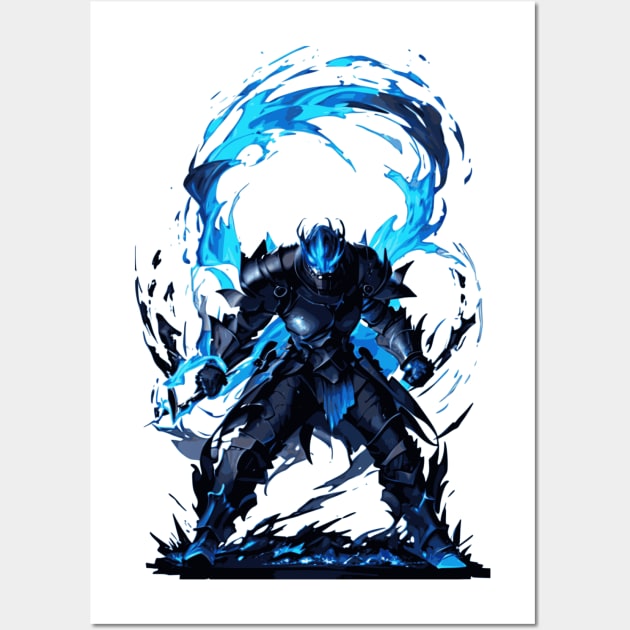The image is a detailed and vibrant digital artwork set on a large white canvas with an off-white, grayish background. It portrays a muscular, menacing, black-suited figure, which resembles a powerful demon or alien warrior from a comic book or video game. The creature has a blue head and shoes and stands ready for combat with its fists clenched, exuding a sense of formidable strength and intimidation. The atmosphere around the figure is charged with dynamic blue swirls or flames that rise from the black, interspersed ground. These blue elements suggest an aura of control over some mystical or elemental force, enhancing the figure's otherworldly presence.